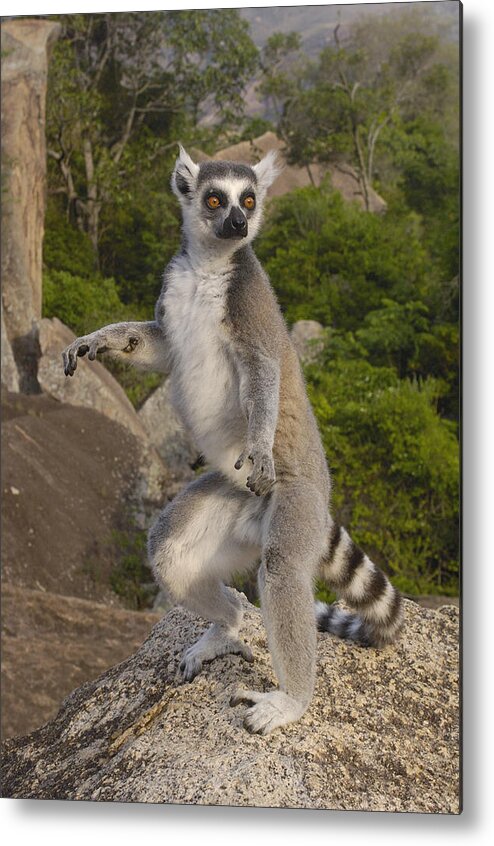In this detailed photograph, we observe a life-sized ring-tailed lemur, possibly a mounted specimen, standing alertly on a rugged, gravelly surface under the bright afternoon sun. The scene is set in a wilderness filled with trees and bushes, framed by distant hills and mountains. The lemur, less than a meter tall, is strikingly posed upright, gripping the ground with its opposable fingers and toes. Its ringed tail, adorned with alternating black and white stripes, trails behind it, touching the ground. The lemur's fur is predominantly gray, with dark and light gradients, while its chest and inner limbs are white. It has a distinctive black snout, wide bright orange eyes with black pupils, and white, pointed ears. Both of its hands are open, with the right arm raised halfway, giving it an attentive and lifelike appearance.